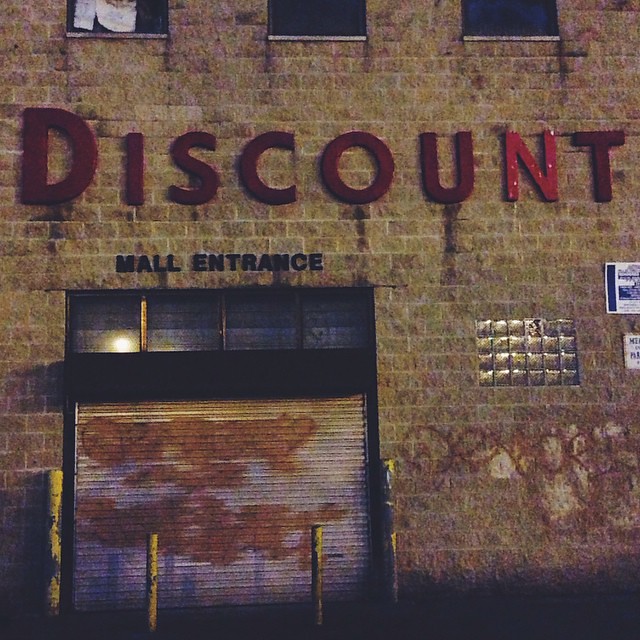This photograph captures an aged brick storefront, its facade marred by a mix of graffiti and weathered stains. The building prominently features the word "DISCOUNT" in large, dark red letters at the top, fading into a brighter red towards the end. Below, "HALL ENTRANCE" is written in bold black capital letters. The structure includes three black windows along the top, each tarnished with long, vertical streaks. Additionally, there's a grid of glass block windows—six across and four down—to the right of a weathered garage door. This silver garage door, accentuated with brown graffiti smudges, is framed by a set of four sturdy yellow poles: two flanking the sides and two directly in front. The overall scene conveys a sense of a once-vibrant location now succumbing to decay and neglect.